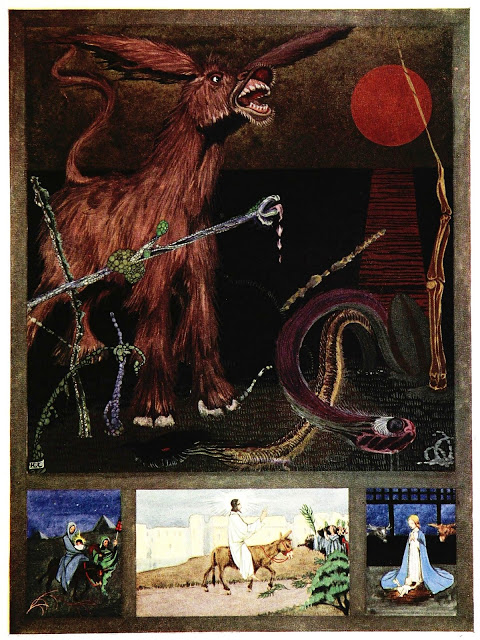The image is a colorful painting divided into four frames, featuring a blend of historical and fantastical elements depicted in a cartoon-like style. The large frame at the top showcases a brown animal that resembles a donkey, barking at a red sun, with a snake positioned to its right. This scene is set against a nighttime backdrop. Below, three smaller frames capture different vignettes. The left frame portrays a young woman, dressed like the Virgin Mary, holding a child with pyramids in the background. The center frame features a person in a white robe, likely representing Jesus, riding a large feline creature or a donkey, flanked by followers. The right frame depicts a woman in a floor-length blue robe standing near two or three hooded figures in a nighttime setting. The image is vibrant without any textual elements, emphasizing the visual storytelling of these interconnected scenes.